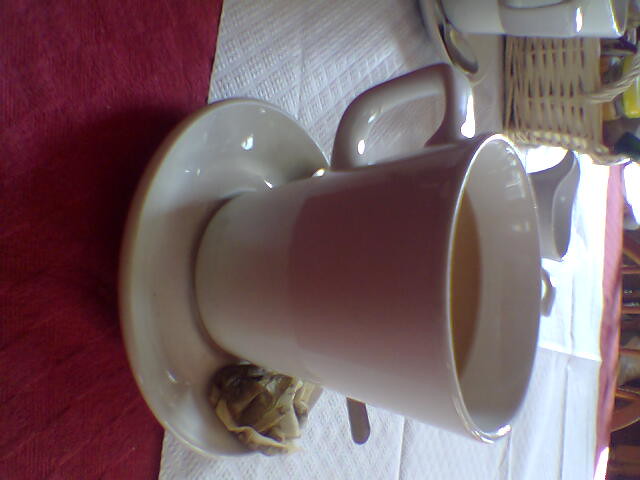This full-color photograph, taken indoors during daytime for artistic purposes, features a white cup on a matching white saucer filled with light brown liquid and a crumpled tea bag at the bottom, suggesting it's tea. The image is oriented sideways, causing the cup's handle to be near the top and the saucer near the left. It rests on a table adorned with a red tablecloth covered by white paper, accented by sunlight streaming through a window. In the background, partially visible, is a white porcelain cream pitcher and a brown wicker basket holding condiments. Additionally, the handle of another cup and saucer set, along with a spoon on the saucer, can be seen in the upper right corner.